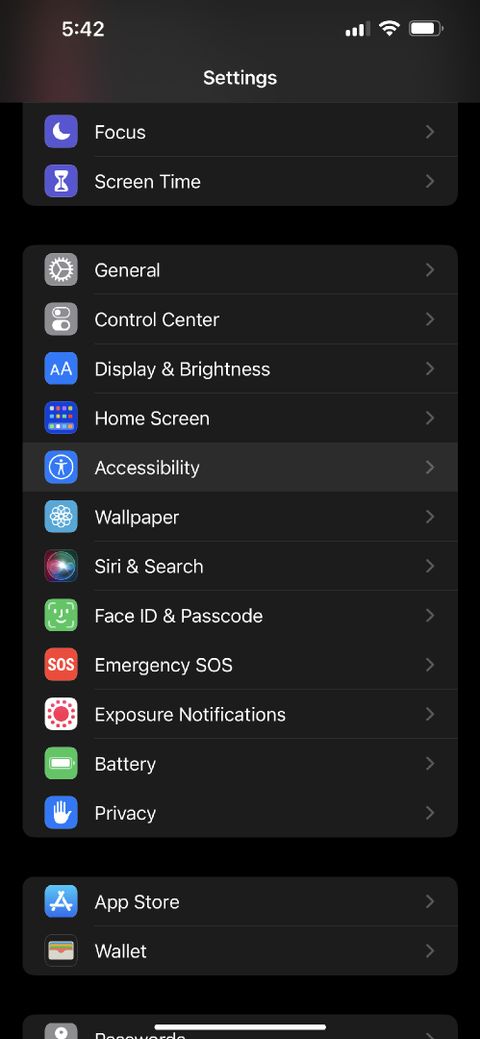A screenshot from a smartphone taken at 5:42 PM displays the device's status bar at the top, indicating full Wi-Fi connectivity, three or four cellular signal bars, and approximately 80% battery life. Below the status bar, centered on the screen, is the word "Sentence." Towards the bottom left, there is a vertical menu. Each entry in the menu is accompanied by an icon on the left and a right-facing arrow on the right, suggesting the availability of drop-down options. The menu is organized as follows:

1. Focus
2. Screen Time

After a small gap, the menu continues with:
3. General (represented by a gear icon)
4. Control Center
5. Display & Brightness
6. Home Screen
7. Accessibility
8. Wallpaper
9. Siri & Search
10. Face ID & Passcode
11. Emergency SOS
12. Exposure Notifications